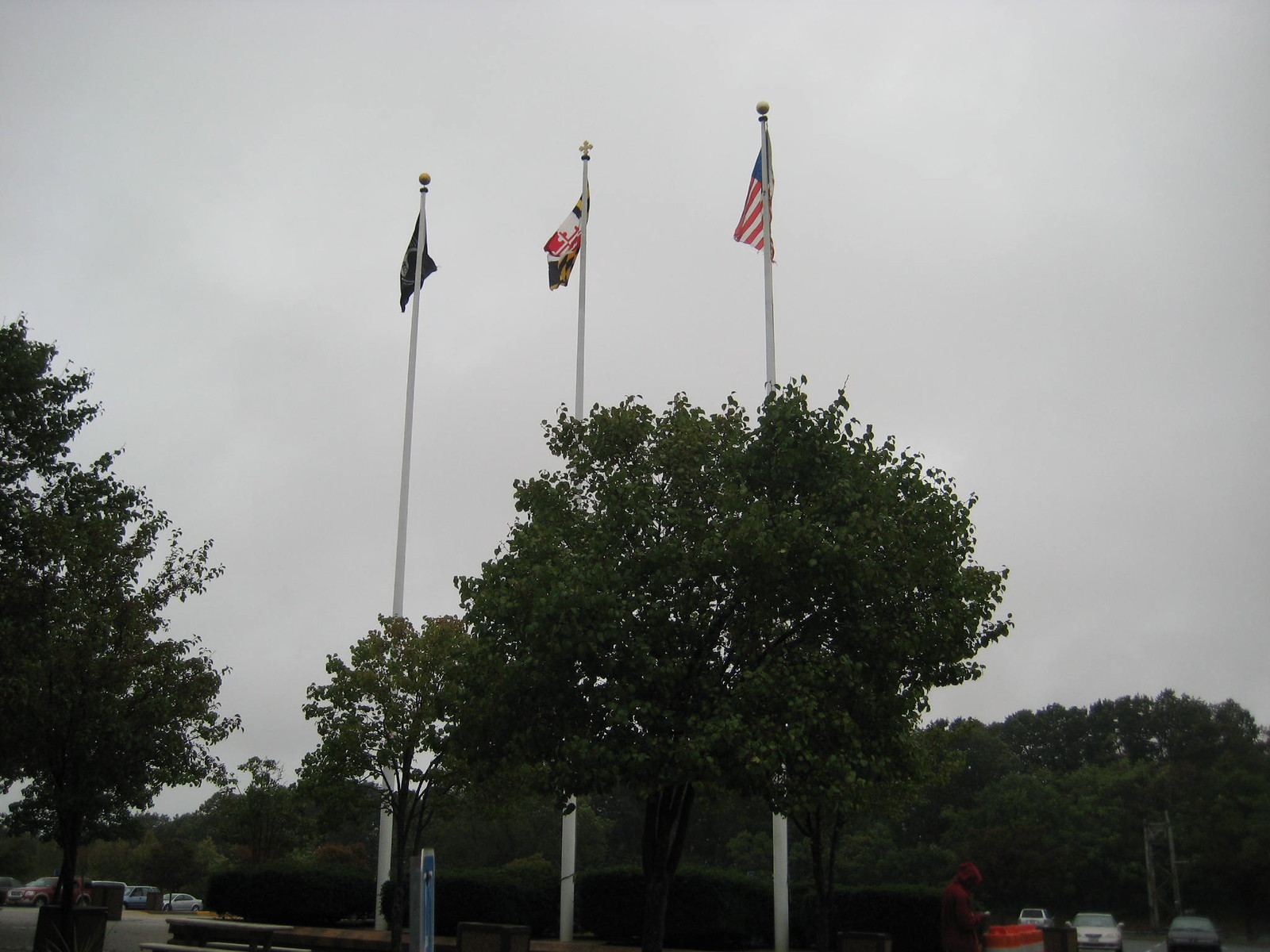In this outdoor photograph, captured on a gloomy, hazy day, three tall white flagpoles rise above a parking lot filled with indistinct cars. The flagpoles, crowned with metal finials, include an American flag on the right, a state or municipal flag in the center, and an unidentified flag on the left. The center pole features a distinctive cross at its peak, suggesting a possible religious significance. Partially obscured by lush, leafy trees that span most of the height of the flagpoles, the flags are lightly fluttering in the gentle breeze. The scene is under a gray sky with scattered clouds, lending a subdued and somewhat colorless tone to the overall image.